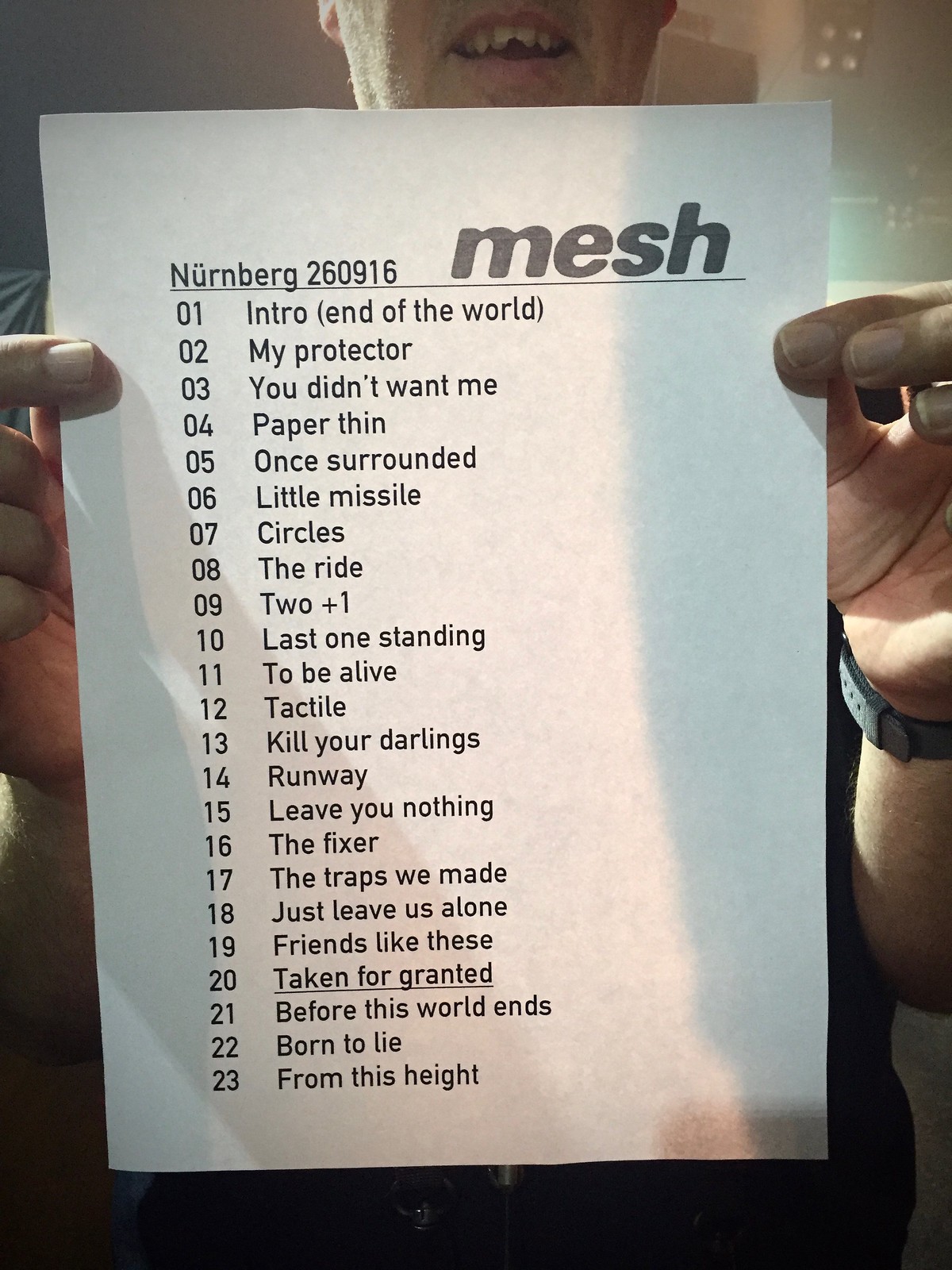The image features a man, partially visible with only his mouth shown, standing in the background while holding up a piece of paper close to the camera. The paper, gripped between his thumb and index finger on both sides, lists what appears to be a concert set list. At the top, it reads "Nuremberg 260916" and "mesh." The list is numbered from 1 to 23, with each number corresponding to a song title. The songs include: 01 - Intro, End of the World; 02 - My Protector; 03 - You Didn't Want Me; 04 - Paper Thin; 05 - Once Surrounded; 06 - Little Missiles; 07 - Circles; 08 - The Ride; 09 - Two Plus One; 10 - Last One Standing; 11 - To Be Alive; 12 - Tactile; 13 - Kill Your Darlings; 14 - Run Away; 15 - Leave You Nothing; 16 - The Fixer; 17 - The Traps We Made; 18 - Just Leave Us Alone; 19 - Friends Like These; 20 - Taken for Granted (underlined); 21 - Before This World Ends; 22 - Born to Lie; and 23 - From This Height. The man appears to be smiling excitedly, possibly indicating his enjoyment or pride in holding this set list.